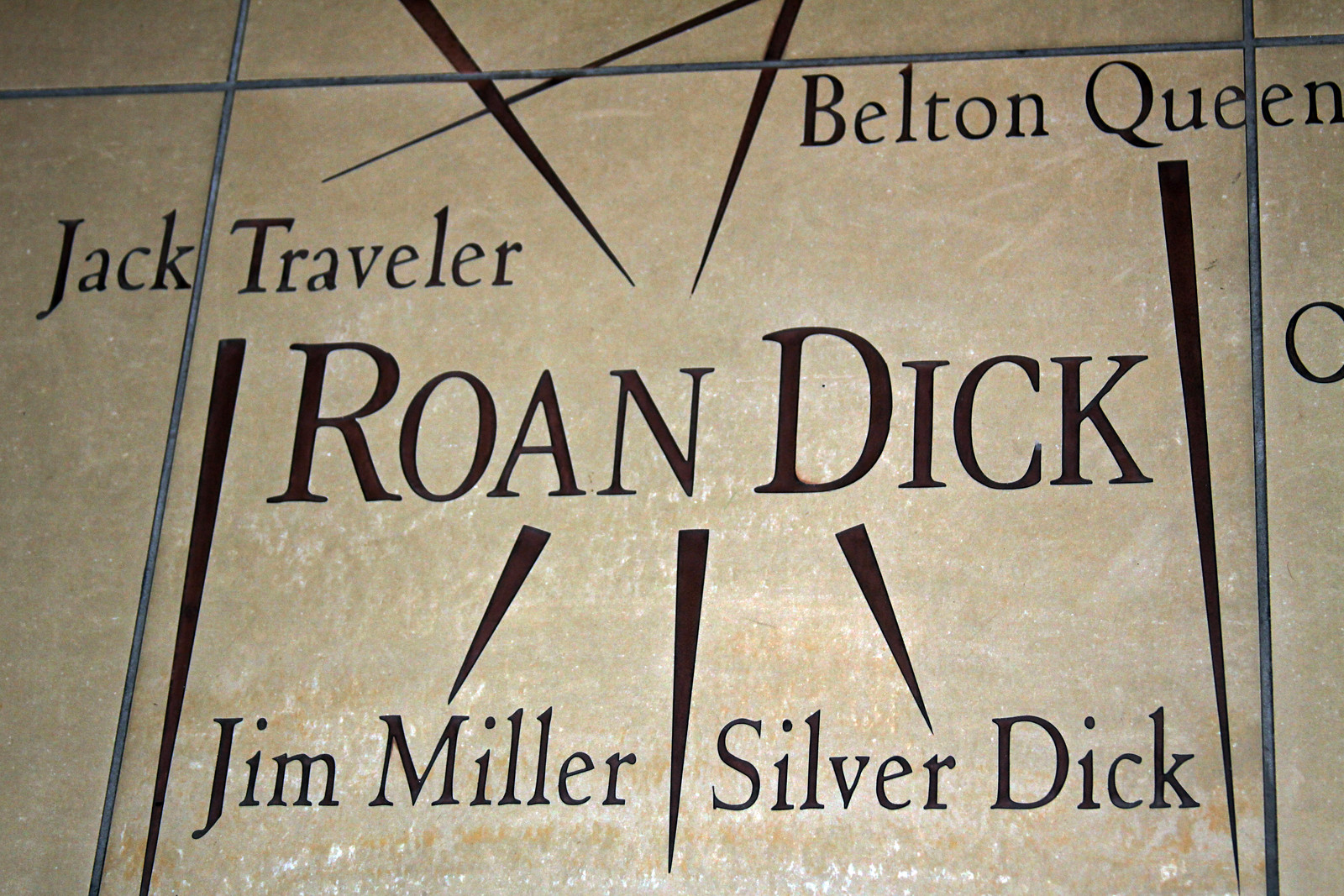A close-up image captures the writing on a textured, beige marble surface with visible gray separation lines between tiles. Prominently in the center, the large brown letters pronounce "ROAN DICK," with several black lines radiating from this central name. These lines vary in direction; one to the left of the 'R' and another starting above the 'K,' both tapering as they extend off the image. Beneath "ROAN DICK," three black lines converge to an end point, each differently positioned: the left line pointing downward leads to "Jim Miller," the middle line acting as a divider, and the right line inclining towards "Silver Dick." Additional names are dispersed across the image: "Jack Traveler" begins to the left of a gray separation line and continues to the right; "Belton" starts above "Queen" at the upper right of the image. The layout appears somewhat chaotic, with names scattered and lines not consistently pointing to other text elements, though they occasionally align. The overall scene resembles an intricate display on tiled marble.